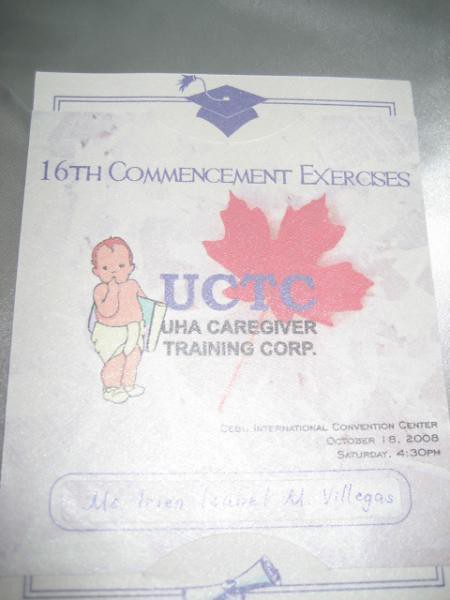The image depicts an official flyer for the "16th Commencement Exercises" of the UCTC, which stands for UHA Caregiver Training Corp. The flyer, set against a gray or silver background resembling stainless steel, is predominantly white with vivid blue accents. At the top of the paper, two horizontal blue lines extend across the page and slightly downward on both sides, framing a blue graduation cap in the center. Beneath this, the following text is displayed sequentially in blue: "16th Commencement Exercises," “UCTC” atop a red leaf, and “UHA Caregiver Training Corp.” Below this, faint and blurred text due to lighting, makes it difficult to read in full, but a blue graduation scroll is discernible. Mentioned clearly in blue are the details: "International Convention Center, October 18, 2008, Saturday at 4:30 p.m." Adding a unique touch, the image also includes a baby wearing a white diaper, holding a blue-and-white notepad, further emphasizing the theme of the 16th Commencement Exercises.